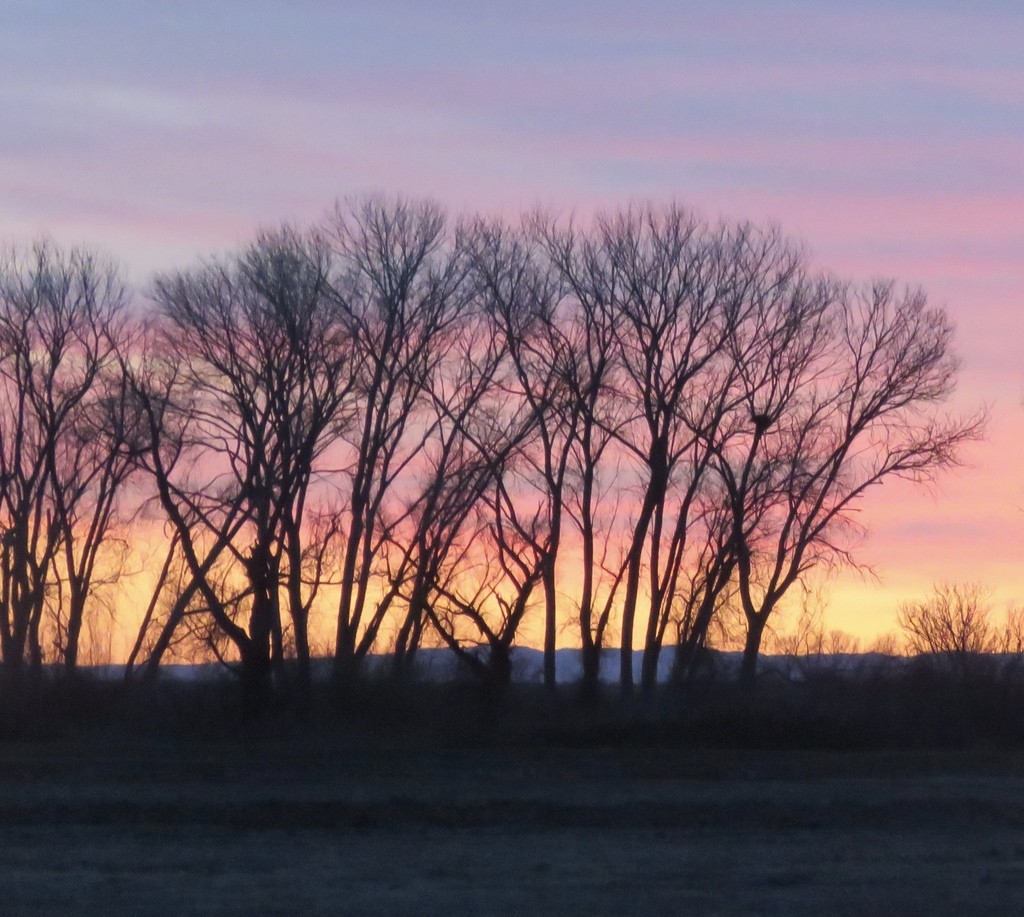This early morning photograph captures a serene and bare scene of nature. The image showcases a field with a dirt-filled foreground transitioning to the distant view of trees lined up from left to right. These trees are completely devoid of leaves, standing tall and starkly silhouetted against a stunning sky. The sky transitions from light blues, grays, and purple haze at the top, blending into pinks and purples, and ultimately fading into a bright, yellowish hue where the sun is rising. In the far distance, snow-capped hills add a touch of rugged beauty. The atmosphere has a dim, haze-like quality that gives the overall scene a tranquil, almost ethereal feel.